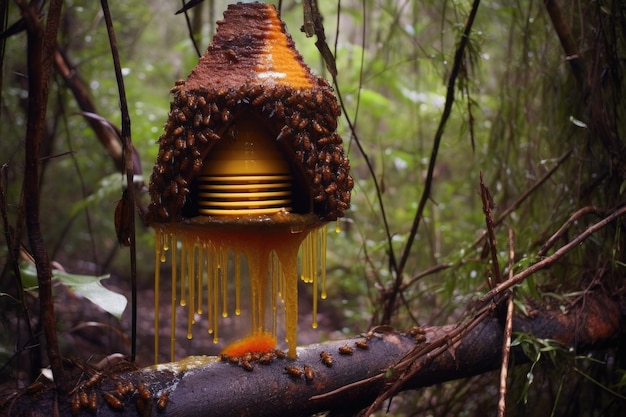In this detailed photograph set in a dense forest filled with trees and vines, a large, lantern-like beehive takes center stage slightly off-center to the left. This beehive, appearing to be a man-made structure possibly constructed from metal or plastic with a distinct core and vent-like features, is covered with swarms of bees closely packed together and working intently. The hive itself is shaped like a cone and is yellow with some brownish substances on top. Thick strands of sticky honey are oozing and dripping from the sides of the hive, cascading down onto a thick branch below. Some bees are dispersed on this branch, seemingly feeding on the dripping honey. The overall scene is somewhat gloomy and dark near the hive but brighter in the distance, where the forest is lush with various broken twigs, branches, and dense vegetation.